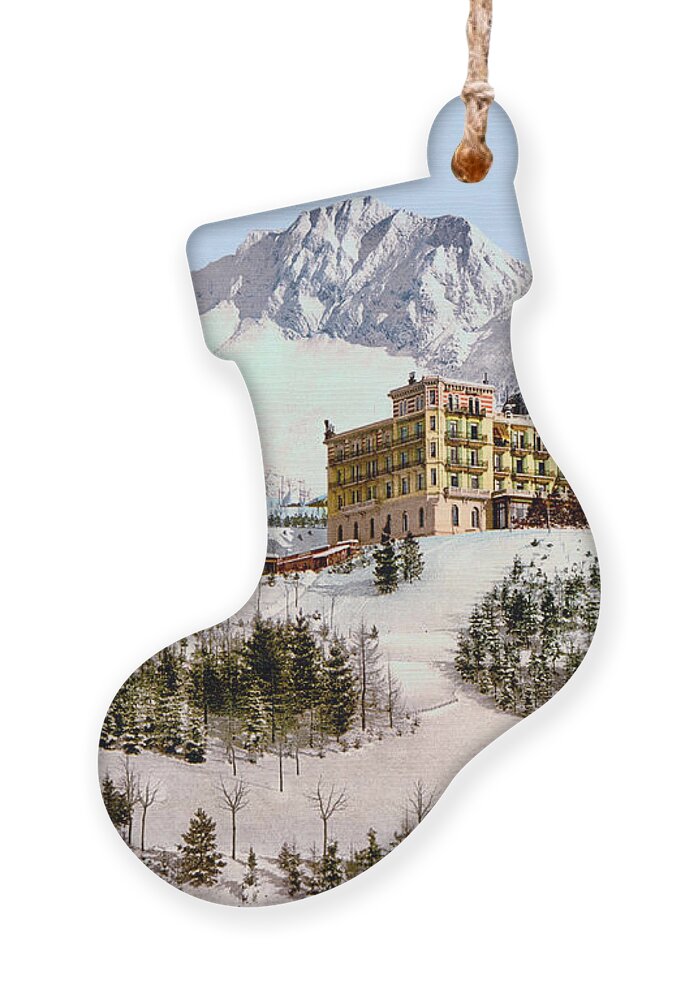This image, presented in portrait orientation, depicts the outline of a Christmas stocking with a photographic scene inside. The stocking shape has a piece of twine at the top, suggesting it is hanging. The toe of the stocking points to the left and the heel to the right. Inside the stocking outline, a snowy landscape is shown. Dominating the scene is a large, possibly four-story, stone-sided building reminiscent of a European ski resort or an old mining town structure, with numerous windows and a beige color. This building sits amidst a winter wonderland, with snow-covered grounds and numerous pine trees surrounding it. The mountainous backdrop features a prominent gray peak, creating a picturesque setting. Scattered around the scene are ski slopes and trails, further emphasizing a winter sports venue. The entire image gives a cozy, festive feel with its Christmas stocking frame holding a serene, snow-filled mountain town scene.